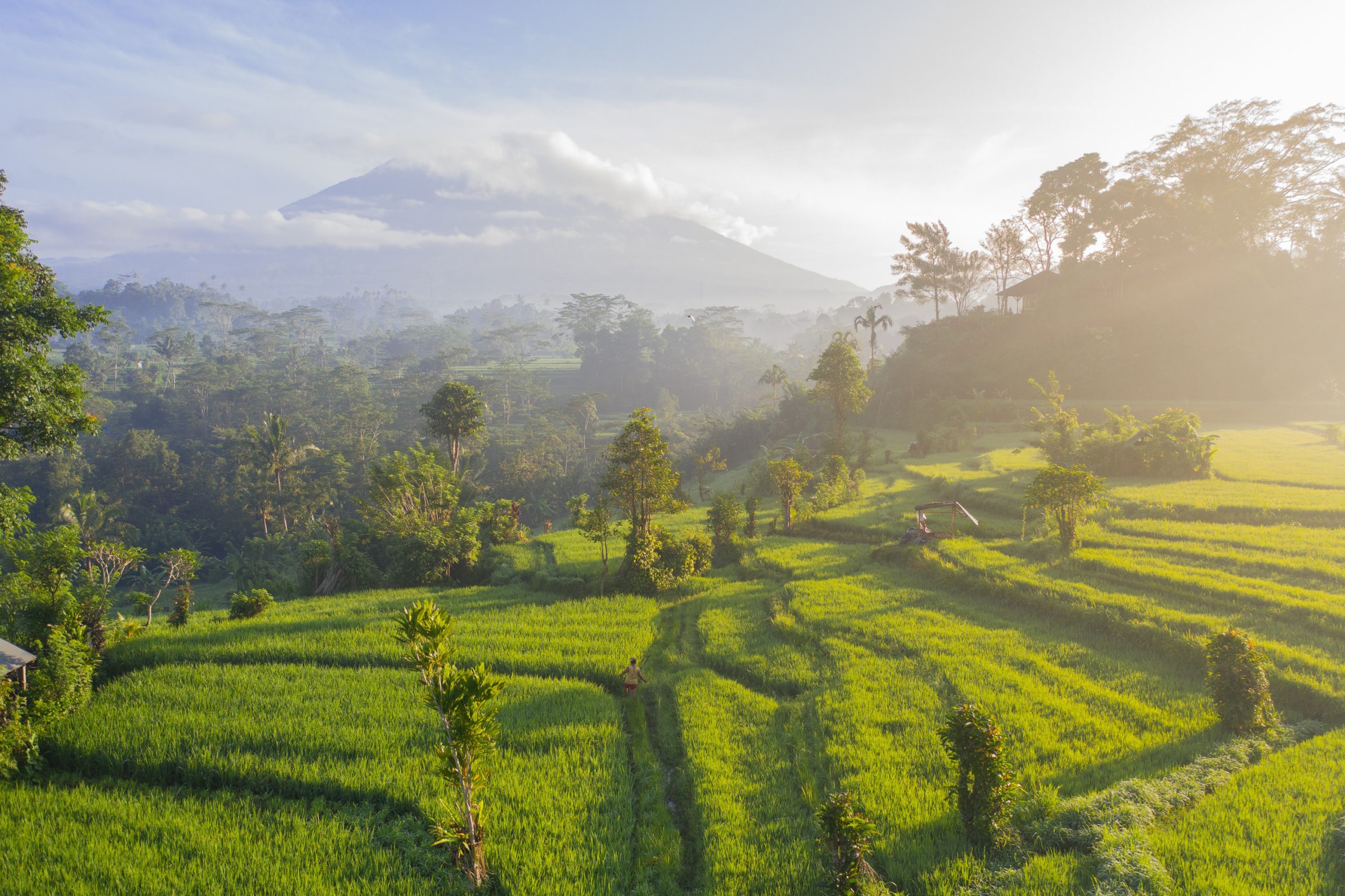This photograph captures a vibrant and diverse landscape. In the foreground, lush, tall grasses dominate the scene, intermixed with various green bushes and trees. A winding path cuts through the greenery, guiding the gaze toward a person walking amidst the grasses; this individual dons yellow clothing and red shorts. On the right side of the image, the sunlight makes the area appear brighter, partially obscuring the colors of the trees with its glare. Towards the far right, a smaller mountain covered with trees emerges, providing a stark contrast to the expanse of foliage. In the distance, a grand, potentially volcanic mountain with a dark, triangular shape looms beneath a blue sky laden with large clouds, ranging from white to gray. To the far left, the dense clustering of trees evokes the sense of a jungle, adding to the image's rich, natural diversity. Adding a quaint touch, a shed-like structure can be spotted among the trees on the right, integrating human presence into this thriving landscape.